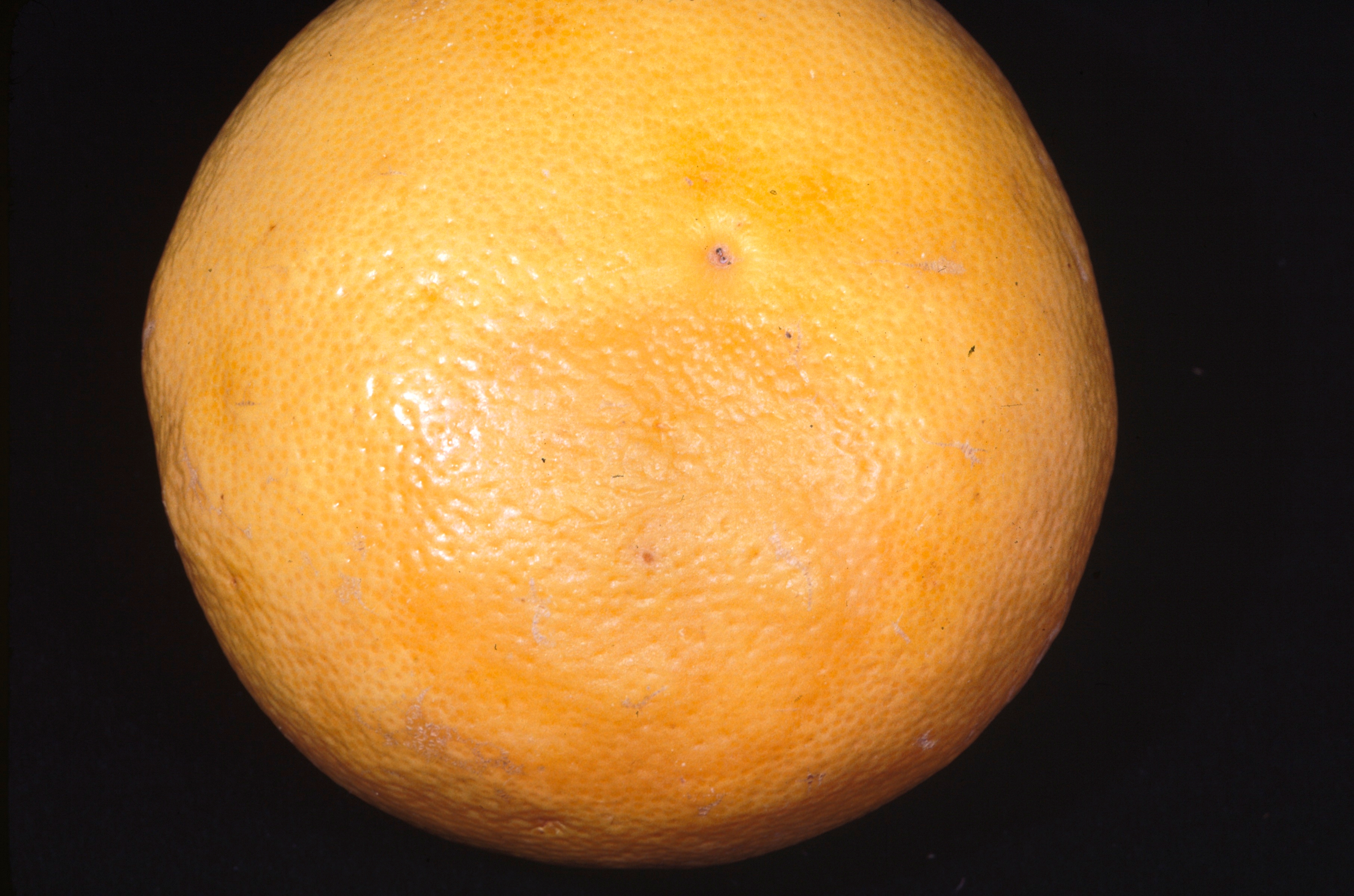This close-up image features a citrus fruit, likely an orange, filling approximately 90% of the frame. The fruit rests against a solid black background, which extends to all sides, emphasizing its prominence. The orange's skin showcases detailed indentations and dimples, reflecting the intricate texture of the rind. The color of the fruit is predominantly bright orange, though it has areas that blend with pinkish and brown discoloration, and some white patches, suggesting it may not be the freshest. Notable is the light reflection on the fruit's surface, indicating the light source is positioned in front. The central section of the orange reveals an indented dimple, adding to its three-dimensional appearance. Overall, the vivid details of the orange contrast starkly with the black backdrop, making it the distinct focal point of the image.